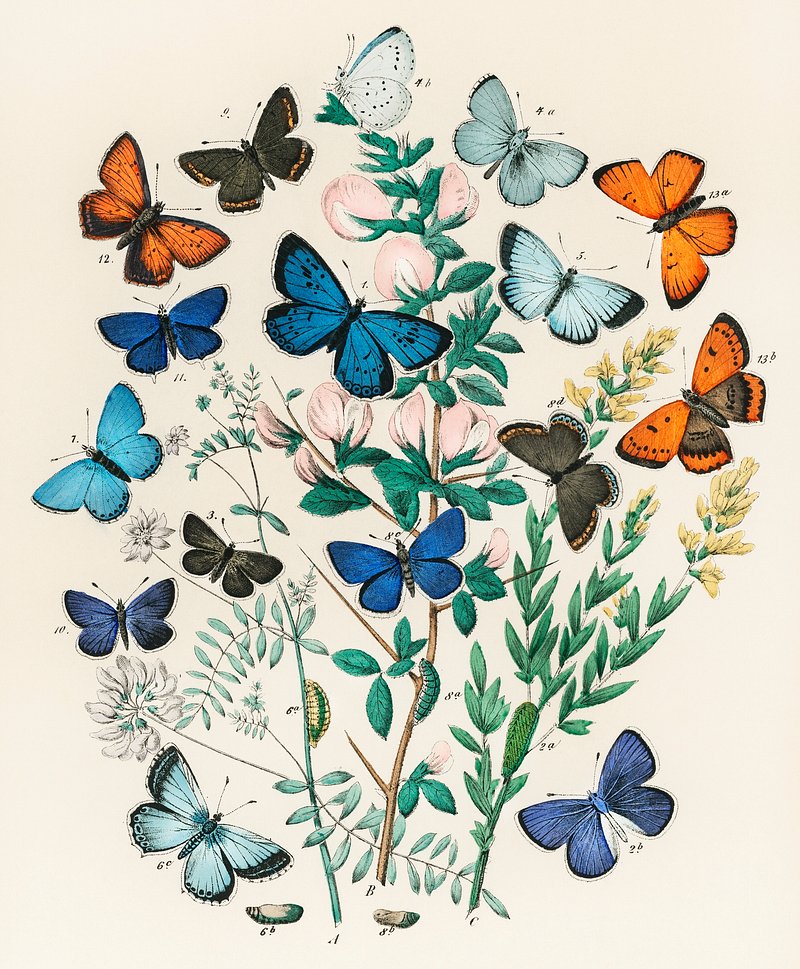This is a vintage color botanical illustration set in portrait orientation, showcasing a variety of butterflies and flowering stems. The central plant features multiple stems with delicate small green leaves and a diverse array of vibrant flowers. The tallest stem in the center is adorned with pink blossoms, while the stems on the right and left display small yellow and white flowers, respectively. The flowers are scattered throughout, with the right stem pointing right and the left stem pointing left. Surrounding the stems is a captivating mix of butterflies, both hovering and perched, rendered in shades of blue, orange, black, yellow, emerald green, and gray. Notable butterflies include monarchs, black with yellow edging, emerald green, light blue, medium blue, dark blue, and a variety with gray and darker gray stripes. At the bottom of the image, several pupae and caterpillars can be seen crawling on the branches, likely on their way to becoming butterflies. Each butterfly is numbered, likely for reference purposes. This detailed watercolor painting captures the delicate beauty and biodiversity of butterflies and flowering plants, reflecting a meticulous vintage style.